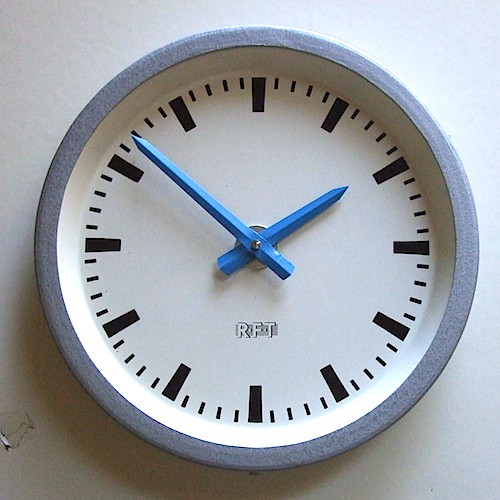A photograph captures a minimalist clock against a stark white wall. The clock hangs slightly off-center, revealing a small, aged piece of tape clinging to the bottom left corner of the wall. The clock's design is simple yet striking, featuring a round white face bordered by a frame in a subdued grayish-blue hue. Instead of traditional numbers, the time is marked by an array of lines and dashes; thicker lines denote the hours, while thinner lines signify the minutes. Underneath the clock's hands, the letters "RFT" appear lightly sketched, reminiscent of a pencil drawing. The clock's hands are a vibrant sky blue, sharply contrasting with the serene backdrop. The time displayed is 2:52. The photo benefits from natural lighting, which streams softly from the top right corner, illuminating the scene without casting harsh shadows.